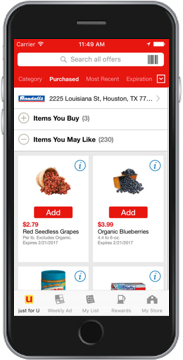This is a detailed description of a cell phone screenshot showing an online shopping app interface. 

The screenshot displays the entirety of the cell phone, including its physical frame. At the top of the screen, there is a red rectangle with several elements. Inside this red banner, a white search bar is prominently centered, containing a gray magnifying glass icon and the placeholder text "search all offers." Situated to the right within the search bar is a UPC code scanner icon. 

Above the red rectangle, the time is displayed at the center, while the upper left corner shows the carrier name and a Wi-Fi signal icon. The upper right corner houses the battery icon. Below this, still within the red rectangle, is a menu bar with multiple tabs. The first tab's label is unreadable, but the second tab is labeled "Purchased" in bold white text, alongside two more tabs with an icon on the far right.

Further down, the background transitions to white. On the left side, a logo is displayed next to an address: "2225 Louisiana Street, Houston, TX 77...". To the right of this address is a light gray arrow pointing to the right. Below this section, a gray-outlined circle contains a gray plus sign at its center. Adjacent to this icon, "Items you buy" is written in bold black text followed by "(3)" in gray parentheses. Underneath, there is another gray-outlined circle featuring a gray minus sign at its center, followed by the text "Items you may like" in bold black with "(230)" in gray parentheses.

The main content area below features two visible squares containing item images, with the tops of two additional squares peeking out from beneath them. Each item square includes detailed information. The first item on the left is red seedless grapes, with an image of grapes at the center. Below the image, a red "Add" button is followed by the price "$2.79" in red text and the product name "Red Seedless Grapes" underneath.

To the right, the next item features organic blueberries priced at $3.99. At the bottom left corner of the screen, the top of a Skippy peanut butter jar is visible, though the item to its right remains unidentified. All items are accompanied by a circle outlined in a light blue line with a lowercase "i" in the center, presumably for additional information.